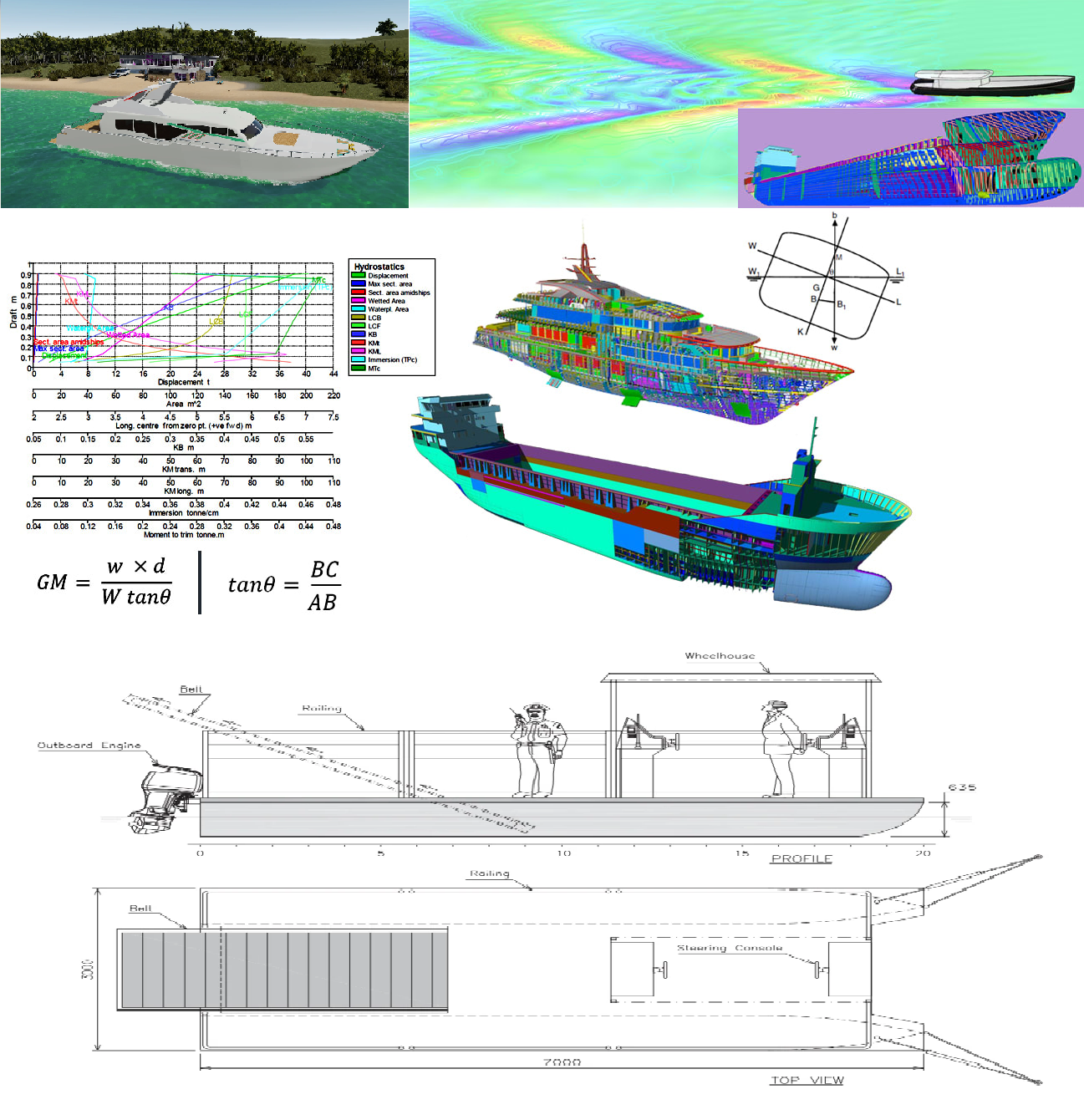This composite image displays a detailed array of boat and ship designs through various mediums. Starting from the top left, there is a computer-generated rendering of a white luxury motor yacht cruising in serene, green waters near a tropical island. Adjacent to it, a working ship navigates through the water with a heat-sensitive image illustrating the turbulence it creates in vibrant colors of blues, oranges, greens, and yellows. An inset within this section reveals another ship, highlighting a unique bow design intended to minimize turbulence. The middle row presents a multi-colored chart labeled with terms like "hydrostatics" and "displacement," accompanied by a cutaway view of two different ships, detailing their internal structures and decks. Below this is a set of pen-and-ink sketches of smaller boats, annotated with technical terms such as "wheelhouse," "outboard engine," and "profile." Mathematical formulas and annotations, including "GM = W x D / W tan θ" and geometric notes, provide additional depth and specificity to the nautical schematics.